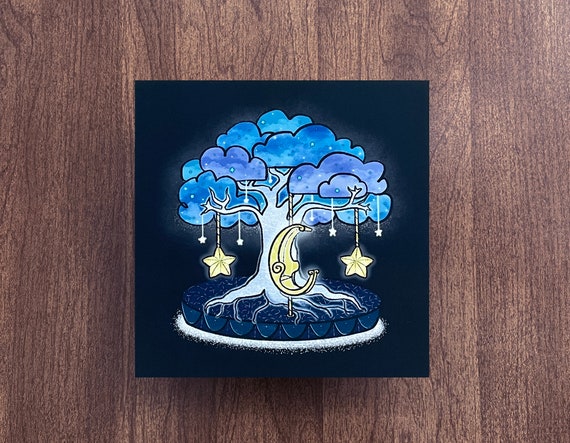This realistic color photograph, horizontally oriented, showcases a striking piece of art against a vertically oriented backdrop of wood panels, likely a wall indicated by the decorative nature of the image. The central square artwork, which resembles stained glass or a detailed reproduction on paper, features a hand-drawn or computer-animated blue tree with a whimsical design. The tree's trunk, branches, and leaves have light and dark blue hues, and the foliage appears as blue clouds. The tree stands on a circular pedestal colored dark blue, surrounded by a ring of white granular material. Beautifully detailed, the branches have strings with stars hanging from them: two medium-sized yellow stars, around seven smaller stars, and a glowing yellow crescent moon prominently in the center, giving it a luminescent quality. The intricate patterns and gentle glow of the moon and leaves lend the artwork an ethereal, dreamlike atmosphere.